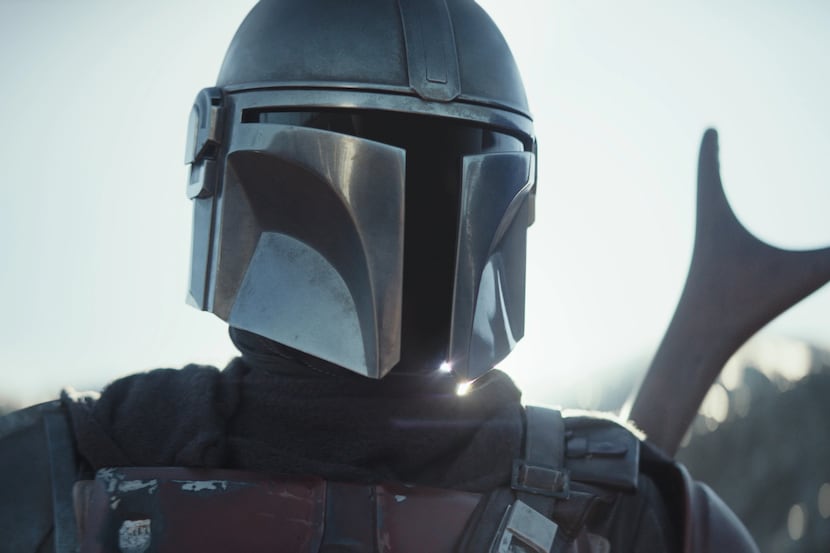In this detailed image of a futuristic space character, the figure is adorned in a full-body suit featuring intricate and modern design elements reminiscent of characters from the Mandalorian in the Star Wars universe. The character's most striking feature is a very shiny, complex helmet, predominantly silver with a darker metal section on the top and front, giving it the classic space helmet appearance. The helmet includes functional hinges on the sides, likely used to lift the face shield. The suit itself is equipped with straps running over the shoulders, secured by a visible metal buckle on the right side. The character appears to be carrying a weapon, possibly a gun, protruding from a pack on their back. The background is dark, contrasting starkly with a very light, almost whitish blue sky that adds an ethereal dimension to the scene.